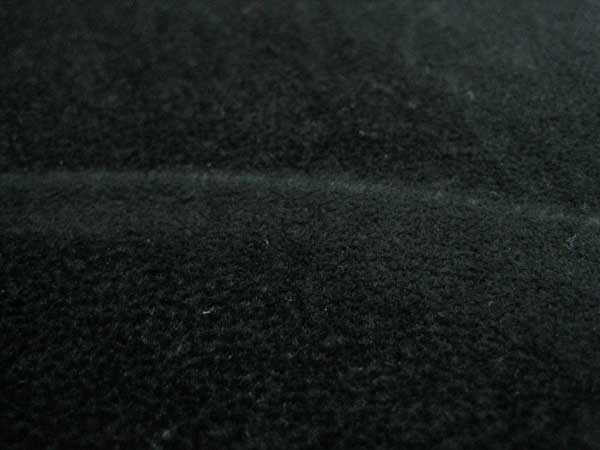The image depicts a highly detailed, close-up view of a blackish-gray, fuzzy texture that resembles the surface of a carpet or perhaps a fleece jacket. The photograph appears to be taken with a macro lens, bringing out the minutiae of the material's fibers. Across the middle of the image runs a themed white curve, which could be interpreted as a seam line. The surface has areas where white patches are visible, suggesting worn-out spots or white dust sprinkled across the material. The entire background is consistent with this black and gray textured appearance, making the white elements stand out distinctly. The lack of any additional objects or text in the photo emphasizes the intricate details and texture of the material captured.